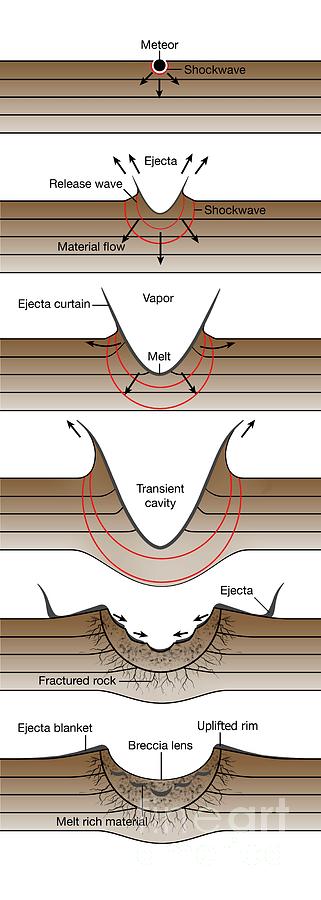This informational diagram illustrates the process and impact progression when a meteor strikes the Earth's surface, depicted through six sequential images stacked vertically. Each image shows the stages of the impact on four distinct brown horizontal layers of the ground.

1. **Initial Impact**: The topmost image shows a meteor, represented as a small black circle, hitting the surface. A line labeled "shockwave" emanates from the meteor, with three arrows pointing downwards diagonally, depicting the initial shockwave's spread.

2. **Ejecta and Release Wave**: The second image continues to highlight the shockwave. It introduces ejecta with three black arrows illustrating material flow, alongside three red concentric rings indicating the release wave's progression downward from the meteor impact point.

3. **Vapor and Ejecta Curtain**: The third image illustrates the expansion of the crater into a V-shape, known as the vapor stage. The crater’s bottom is marked as a melt, with an ejecta curtain forming upwards. Two red lines beneath the crater indicate deeper material displacement, with black arrows showing the movement of materials outwards.

4. **Transient Cavity Formation**: The fourth image presents a deeper and wider V-shaped crater, termed the transient cavity, with arrows emphasizing the outward curvature of its sides. Two red lines beneath suggest extensive subsurface impact, and the crater bottom shows a bulging effect.

5. **Formation of Fractured Rock and Ejecta**: The fifth image shows the transient cavity collapsing slightly into a ruffled crater with scalloped edges and fissures. Labeled as fractured rock and ejecta, this stage includes visual cues of cracks and arrows pointing to the disrupted layers.

6. **Creation of the Ejecta Blanket and Uplifted Rim**: The last image depicts the final impact stage, where the crater has a sloped and elevated rim called the ejecta blanket, with the bottom layers showing both fractures and small holes termed as the brachial lens. This phase also indicates the presence of melt-rich material.

Overall, this detailed vertical sequence effectively captures the dynamic and transformative effects of a meteor impact on the Earth's stratified surface layers, from initial impact through to the final crater formation.